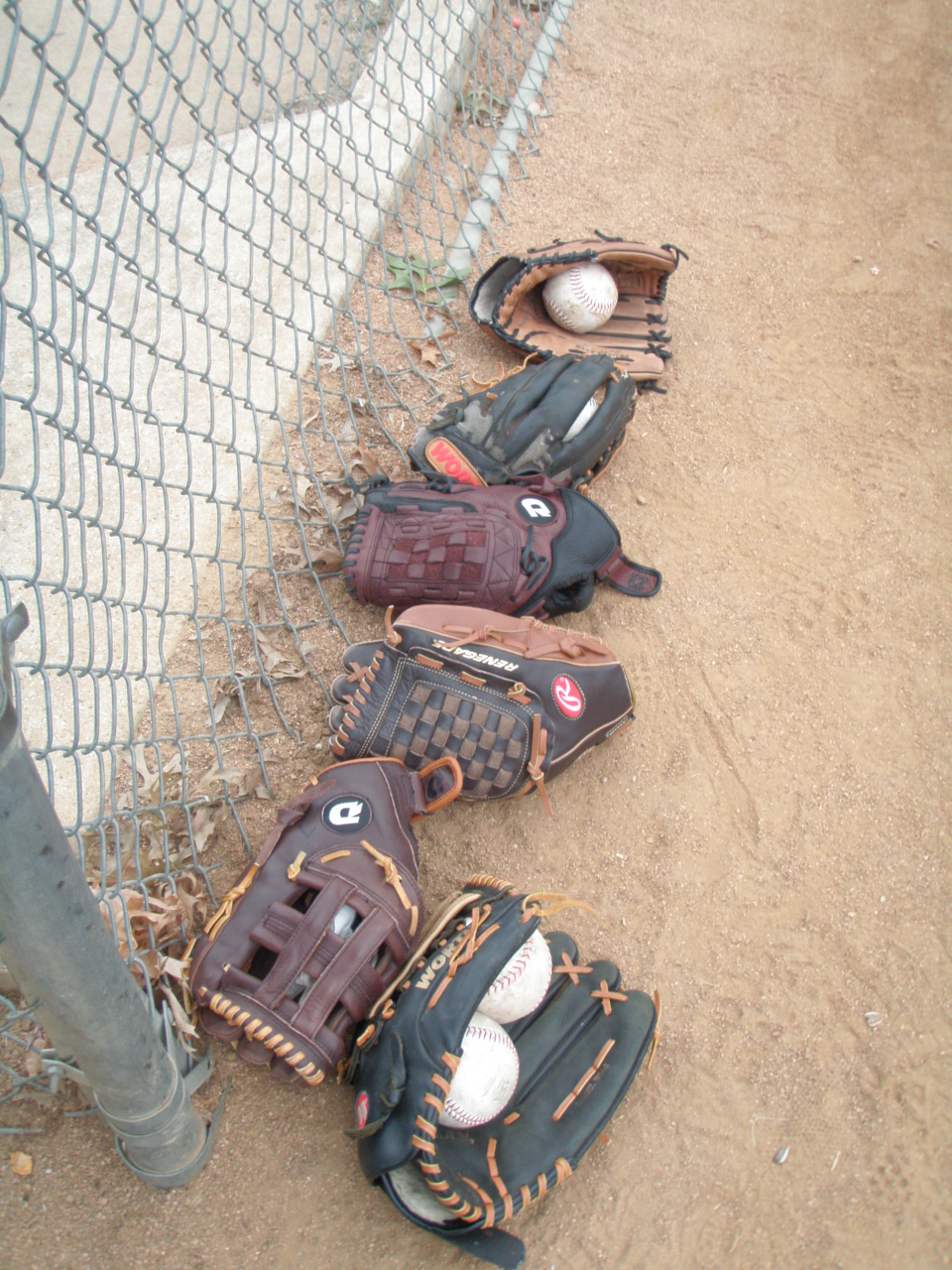The image is a color photograph taken outside during the daytime, capturing a close-up view of six baseball gloves arranged on a dark brownish sandy surface, likely in a baseball field area. These gloves, varying in colors and styles, include black, tan, and different shades of brown with varied lacing in orange, russet, and tan hues. Some gloves also feature distinctive logos and initials, such as a black glove with tan lacing and a "W," and another with a "P" inside a red circle.

Nestled inside several of the gloves are pristine white baseballs adorned with the iconic red U-shaped stitching. The gloves and balls are positioned against a chain link fence, which runs along the left side of the image. The metal fencing appears slightly bowed, indicating some damage, and extends upwards out of the image diagonally towards the back right. 

In the foreground, the base of the fence post is visible, partially buried in the sand. Beyond the fence, the ground transitions into a light tarmac area scattered with a mix of light and dark brown leaves, as well as some green foliage. The detailed layout and varied elements in the frame contribute to a rich, textured depiction of a typical scene from the peripherals of a baseball field.